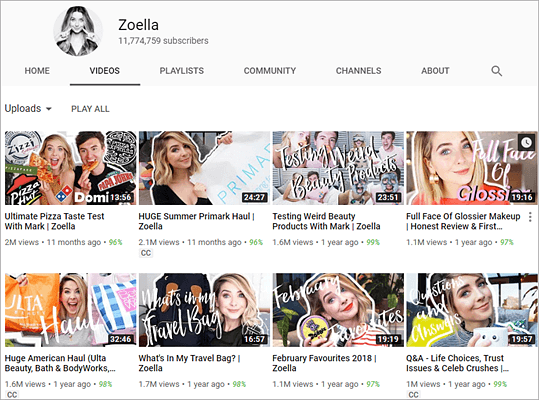This image is a screenshot of Zoella's YouTube channel interface, capturing a detailed snapshot of her page. In the upper left-hand corner, her profile picture is displayed within a circular frame. Adjacent to her profile picture, the channel's impressive subscriber count is shown, standing at 11,774,759. The top navigation bar spans horizontally across the page with tabs labeled Home, Videos, Playlist, Community, Channels, and About, providing easy access to different sections of her channel.

The main content area of the screenshot features a grid of eight video thumbnails, organized in two rows of four. Zoella appears in all the video thumbnails, primarily in headshots. In the first and third videos, she is seen alongside a person named Mark. Additionally, in several of the thumbnail images, she is holding up various items, presumably related to the video content. The visual layout and strategic organization of her content provide viewers with an inviting and well-structured interface to explore her videos.